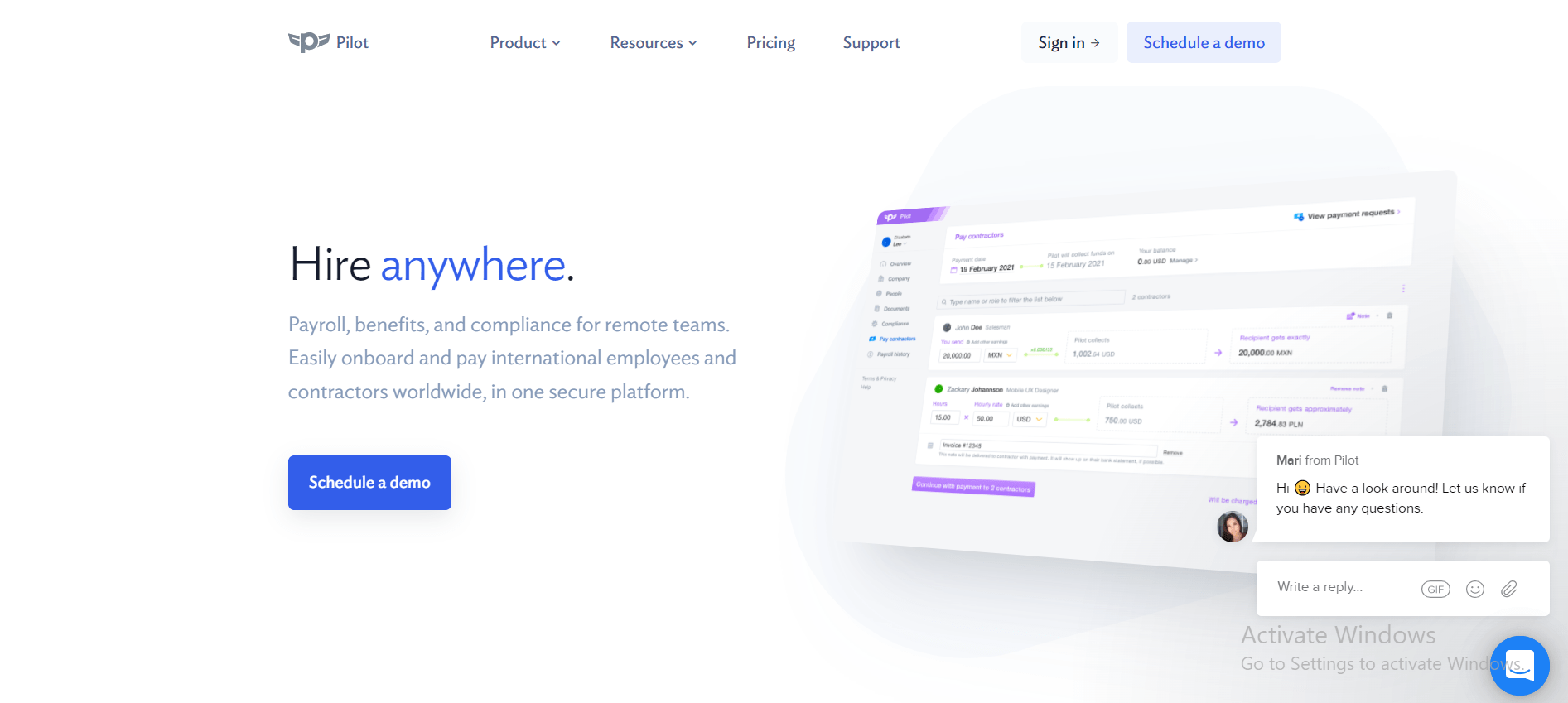This is a cropped screenshot of the homepage of the Pilot website. At the top left corner, the Pilot logo is displayed in gray. To the right of the logo, the navigation menu includes four categories: Product, Resources, Pricing, and Support. The Product and Resources categories feature drop-down boxes. On the far right, there are two buttons: "Sign In" and "Schedule a Demo." The "Schedule a Demo" button is blue with blue text. The background of the webpage is white.

Towards the center left, the text "Hire Anywhere" is prominently displayed, with "Hire" in large black font and "Anywhere" in lowercase blue font. Below this, in small blue letters, it says, "Payroll, Benefits, and Compliance for Remote Teams. Easily onboard and pay international employees and contractors worldwide in one secure platform." 

Further down, on the left side, there is another "Schedule a Demo" section with a blue button also labeled "Schedule a Demo." To the right side of the image, an angled view of a spreadsheet is shown, with a chat box overlaid at the bottom right corner. The chat box features a profile photo in a circle at the bottom left and the name of the sender at the top. The message reads, "Hi 😊 Have a look yourself and let us know if you have any questions." Below this message, there is a "Write a Reply" box. Additionally, there is a blue circle with a chat icon at the bottom left of the chat box.